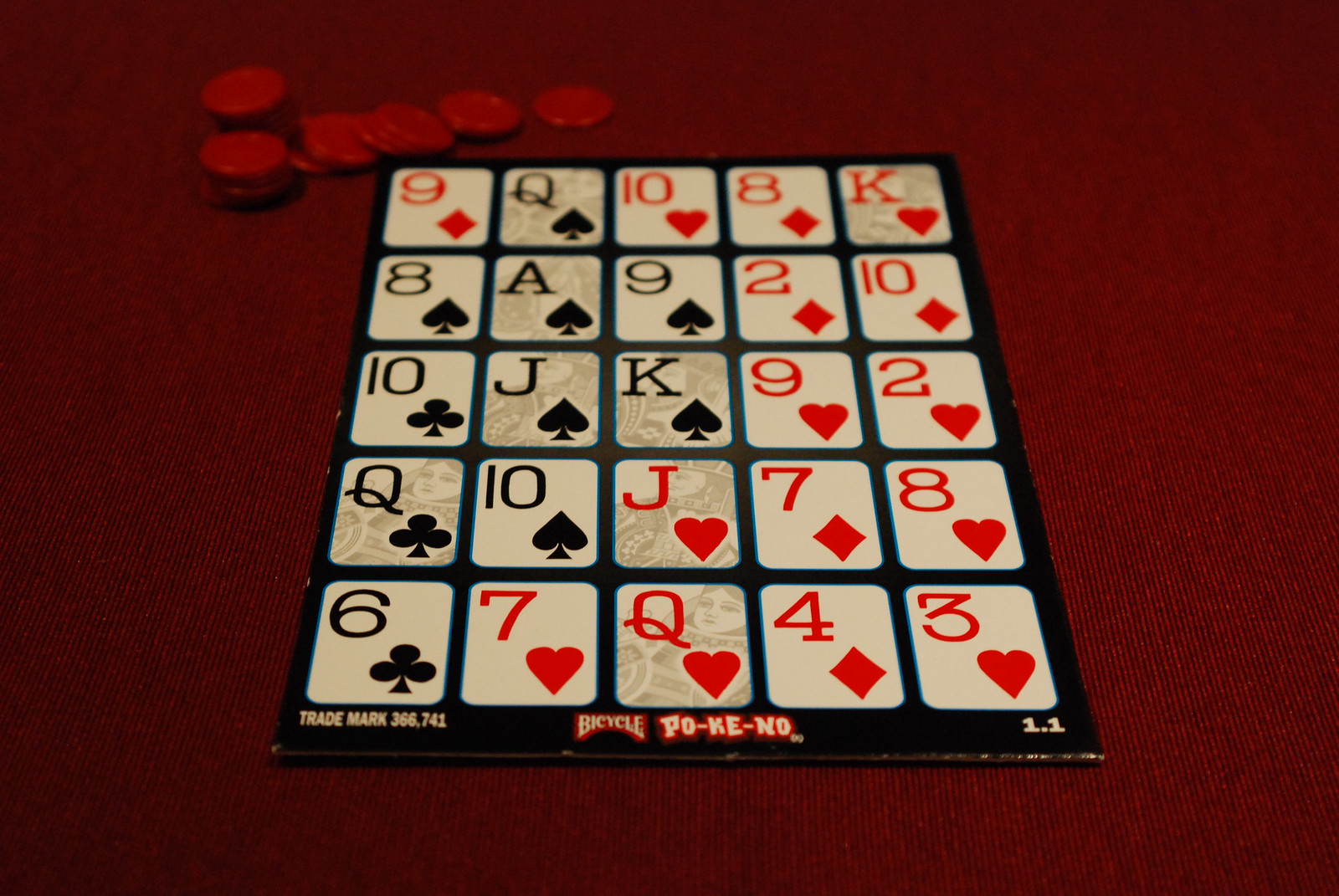The image is an indoor color photograph taken from above, displaying a grid of playing cards organized in five rows and five columns. Each card shows various face values from a standard deck. In the upper-left corner, there is a stack of approximately 20 red poker chips, some forming two small piles while others are scattered nearly in a horizontal line. The surface under the cards and chips is a vibrant, wine-colored cloth.

Focusing on the grid of cards, the first row (left to right) contains the following: a red Nine of Spades, a black Queen of Spades, a red Ten of Hearts, a red Diamond, and a red King of Hearts. The second row includes: a black Eight of Spades, a black Ace of Spades, a black Nine of Spades, a red Two of Hearts, and a red Ten of Diamonds. The third (center) row displays: a Ten of Clubs, a Jack of Spades, a King of Spades, a red Nine of Hearts, and a red Two of Hearts. The fourth row consists of: a Queen of Clubs, a Ten of Spades, a Jack of Hearts, a Seven of Diamonds, and an Eight of Hearts. The fifth (bottom) row shows: a Six of Clubs, a Seven of Hearts, a Queen of Hearts, a Four of Diamonds, and a Three of Hearts.

In the lower-left and lower-right corners, the text "Trademark 366.741" is visible. The center of the table features the word "BICYCLE," followed by the term "PO-KE-NO" in hyphenated form. To the right of this, the number "1.1" is inscribed in very small font.